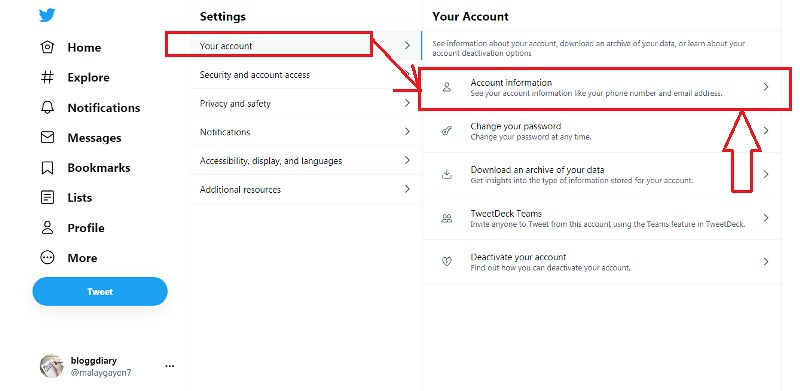Here is a detailed and cleaned-up caption for the described image:

---

The image is a detailed guide for navigating to the Twitter settings page. It starts from the top third of the page, showcasing the Twitter icon situated in the top-left corner, below which are various navigation options aligned vertically. Each option is accompanied by an icon and labeled accordingly. The first option features a small house icon labeled "Home" in black lettering, followed by a pound sign labeled "Explore," a bell icon for "Notifications," and additional options including "Bookmarks," "Lists," "Profile," and "More."

At the bottom of this navigation column, there is a prominent blue button labeled "Tweet." In the bottom-left corner, the Twitter handle "blog_diary" is visible, albeit faintly.

The middle section of the page emphasizes the "Settings" option, highlighted with a red border. Under "Settings," there is a category labeled "Your Account," also bordered in red, displaying six additional options. An arrow points to the right section.

The right third of the image focuses specifically on the "Your Account" section, which is expanded. Within this section, a red-bordered area highlights "Account Information," listing details such as email and phone number.

A large red arrow, filled with white, points upwards towards a rectangular element. Below this, four more options are listed without any highlighting: "Change Your Password," "Download an Archive of Your Data," "TweetDeck Teams," and "Deactivate Your Account." These options provide various settings related to your account management on Twitter.

---